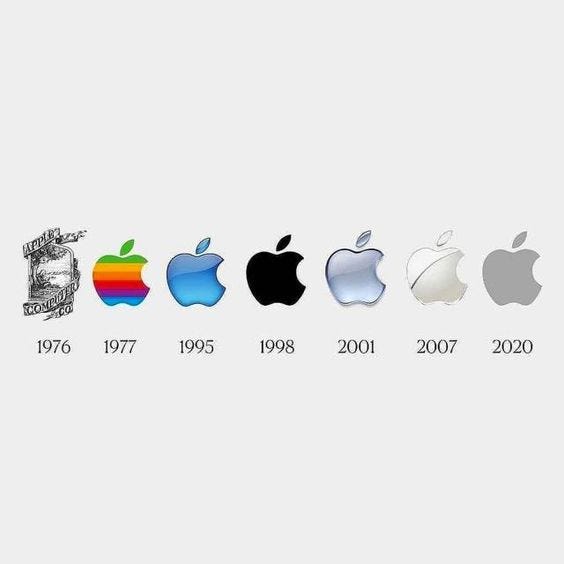The image illustrates the evolution of the Apple logo from 1976 to 2020 against a white background. The timeline begins on the left with the original 1976 logo featuring a detailed, black-and-white pencil sketch of a ribboned banner reading "Apple Computer Co." Moving to 1977, the classic bitten Apple logo appears in rainbow colors. By 1995, the logo transitions to a blue gradient. The next major change occurs in 1998 with a sleek black version of the bitten Apple. In 2001, the logo becomes a striking chrome light blue. The 2007 iteration showcases a minimalist white design. Finally, in 2020, the logo adopts a simple, modern gray tone.